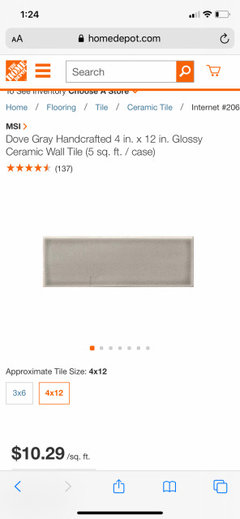Screenshot of a mobile device in portrait mode displaying a website. 

At the top left corner, the time reads "1:24," and the top right corner shows the battery level at approximately 25%. Below this is the browser's URL bar with the address "homedepot.com," alongside a padlock icon indicating a secure connection, and the option to refresh the page.

Following this, the Home Depot logo is prominently displayed, accompanied by three horizontal orange lines representing a menu icon, a search bar, an orange search icon, and a shopping cart icon, all aligned from left to right. A thick orange line runs horizontally across the screen beneath these elements.

Below the orange line, partially obscured text appears to reference inventory with a prompt to choose a store location, displayed above a breadcrumb navigation path that reads: "Home > Flooring > Tile > Ceramic Tile > #206."

The main content area features a product listing for "MSI Dove Gray Handcrafted 4-inch by 12-inch Glossy Ceramic Wall Tile (5 square feet per case)." It has a rating of four and a half stars from 137 reviews. The product image shows a dark gray tile. Below the image, an orange circle indicates it’s one out of seven pictures available.

The text further includes an option to select the tile size with a preference for "4 by 12" inches already chosen, priced at $10.29 per square foot.